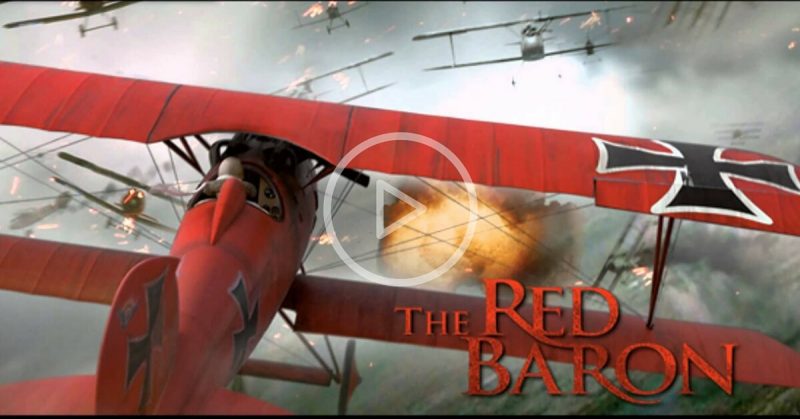The image is a detailed still from a video, likely promoting a movie or featured on a streaming service due to its sophisticated user interface. The focus is on the Red Baron's iconic bright red biplane, prominently marked with black crosses outlined in white on the wings, fuselage, and tail. This biplane is engaged in an intense aerial battle, surrounded by several other metallic gray planes. The chaotic scene includes visible tracers from machine-gun fire, with some planes catching fire and one engulfed in a ball of flames. Explosions in bright yellow and orange hues add to the wartime chaos. The scene is set against a backdrop of dark, thick clouds, with minimal light filtering through, adding to the dramatic atmosphere. At the bottom of the image, the title "The Red Baron" is displayed in all caps with a sophisticated font, emphasizing the film's focus on this legendary pilot.